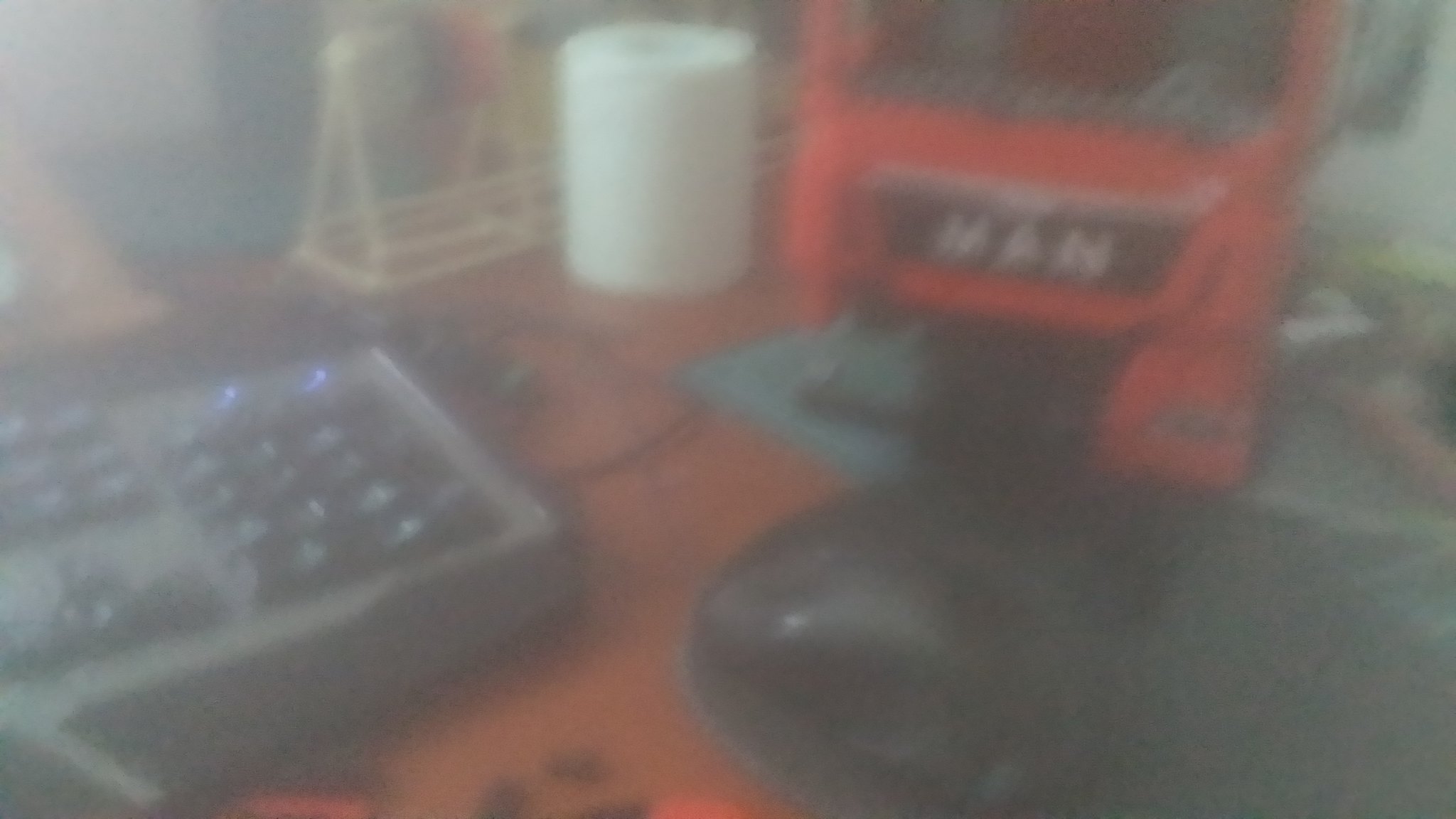This is an extremely blurry and out-of-focus photograph, possibly due to a smoky room or a dirty camera lens, making the scene difficult to decipher. The image appears to capture a brown desktop surface. In the lower left corner, there is a black and gray keyboard featuring black keys and blue LEDs. Above the keyboard, there is a rack for holding papers or magazines, and beneath the rack, a white candle is visible. Central to the image is a red machine with a small black plaque on the front, displaying the word "MAN" in white letters. In front of the red machine, there seems to be a small padded seat. A gray control panel with buttons and lights sits atop what might be a workbench, suggesting a utilitarian workspace. In the background, you can discern a roll of paper towels and a yellow rack, although details are challenging to make out due to the photo's poor quality.